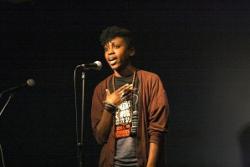In this evocative color photograph, an African American woman with short, pixie-cut hair stands on a dimly lit stage, illuminated by a single spotlight. She is positioned in front of a microphone with a black handle and with a silver top mounted on a stand, her left hand tenderly placed over her heart. Her expression is deeply emotional, as if she is in the midst of delivering a stirring song or spoken word piece. She wears a dark t-shirt featuring indiscernible white and red graphics, layered beneath a brown cardigan with its sleeves rolled up to her elbows. Her wrist is adorned with several dark bracelets, adding subtle detail to her appearance. The surrounding scene is completely dark, drawing all attention to her poignant performance. Another microphone stand, unoccupied, stands to her left. The focus of the image is slightly soft, lending a dream-like quality to the moment captured.